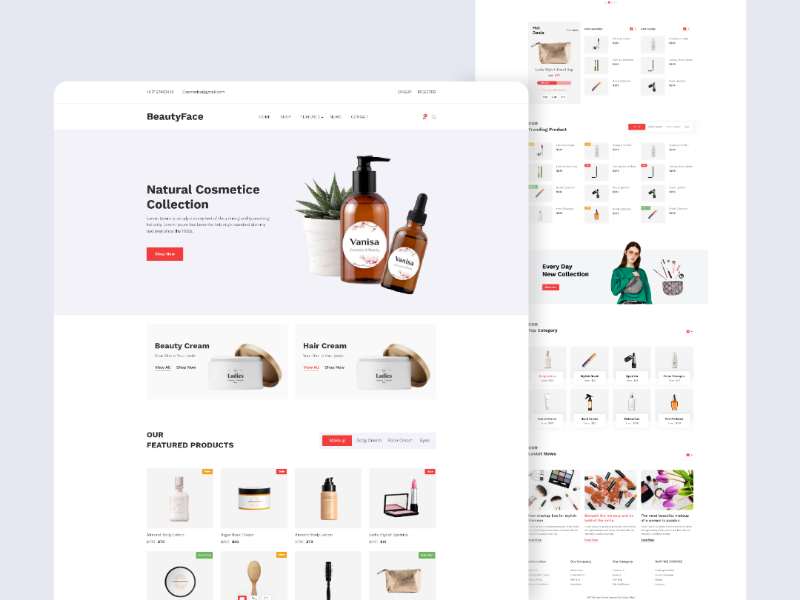The image depicts an interface with a gray border spanning the top and both sides. Dominating the gray area is a prominent window. Although the text within the window is mostly blurry, certain words are discernible: "Beauty," "Face," "Home," "Shop," "Register," and the phrase "Natural Cod Metisque Collection." Below this text lies a red button and an unreadable paragraph. Centrally featured is a white flowerpot containing a plant resembling aloe vera. Accompanying the plant are two brown bottles, both bearing an oval white label with illegible text. The left bottle is equipped with a push pump, while the right one has a dropper. Beneath these items, the words "Beauty Cream" are followed by an image of a small container with a round gold lid. Additionally, a similar container labeled "Hair Cream" is showcased. Finally, the section is concluded with the phrase "Featured Products."